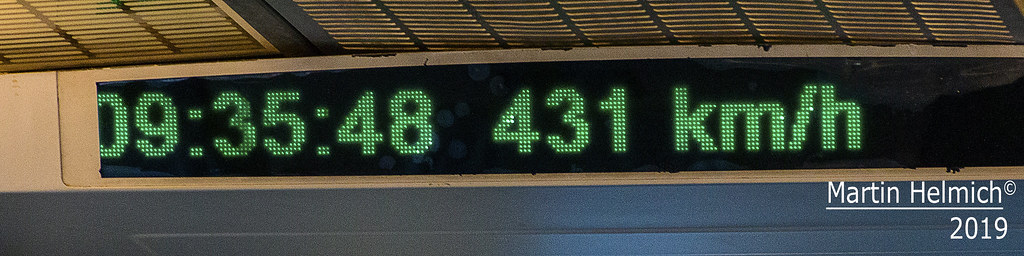Image Description: The photograph captures a horizontal, rectangular digital display sign set against a black backdrop. Illuminated in bright green digital lights, the sign displays the time "09:35:48" followed by the speed "431 KM/H", indicating kilometers per hour. The background and edges of the image reveal the sign mounted on or against a wall. In the bottom right corner of the image, the copyright mark of "Martin Helmich" is visible, clearly denoted with the © symbol next to his name. A white line is drawn underneath his name, followed by the year "2019".